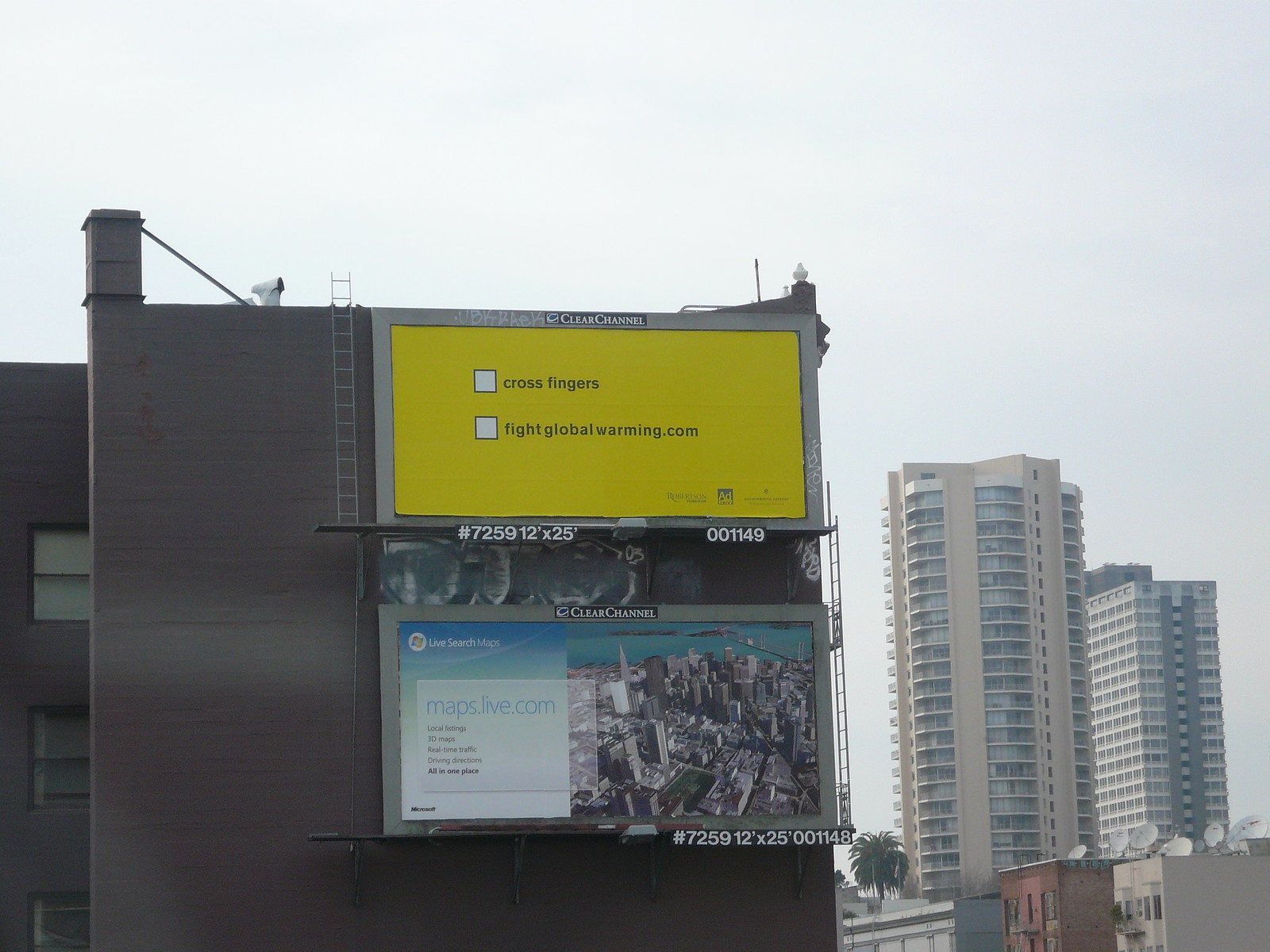This outdoor daytime photograph, taken in bright yet hazy light, prominently features two rectangular billboards mounted on the left side of a five- or six-story all-brick building with a few windows in its lower left section. The top billboard, slightly left of the image center, stands out with its yellow background and two white, unchecked checkboxes. Adjacent to the first checkbox, it reads "cross fingers," while beside the second checkbox it states "fightglobalwarming.com." Additional numbers "#7259 12 by 25 feet" and "001149" are visible on a horizontal walkway in front of the billboard. Below it, the second billboard showcases an aerial cityscape photograph with an overlay in blue lettering saying "maps.live.com," albeit some unclear smaller text. Numbers "#7259 12 foot by 25 foot 001148" appear on a placard hanging from the lower right corner of this billboard. In the photo's background to the right, two towering, white apartment complexes loom, contrasting with some lower buildings visible in the foreground. The sky is dense and gray, conveying a foggy urban atmosphere.